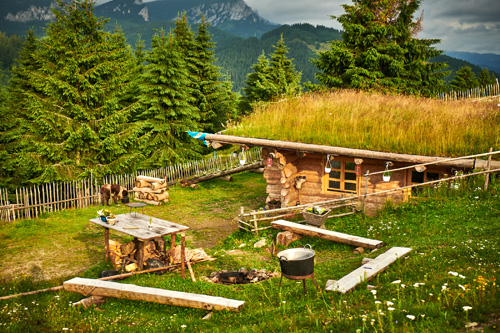This is a detailed color photograph of a serene forest and countryside scene. Dominating the image are tall, densely-packed pine trees with a palette of light green and greenish-brown hues. Nestled into a grassy hill, a quaint, old-fashioned wooden hut captures attention. The hut’s roof, partly embedded into the hillside, is covered with a mix of grass, resembling straw with burnt orange-yellow and green streaks. This structure, with its log construction and yellow-trimmed windows, exudes a rustic charm. The foreground displays scattered logs and a stand with a pot, and possibly a cow or large dog near the cabin. In the background, a range of grayish-blue mountains looms, capped with a touch of snow, while the sky above is partly blue with swirling gray clouds, adding a dramatic touch to this picturesque landscape. White flowers dot the green grass, enhancing the bucolic atmosphere.